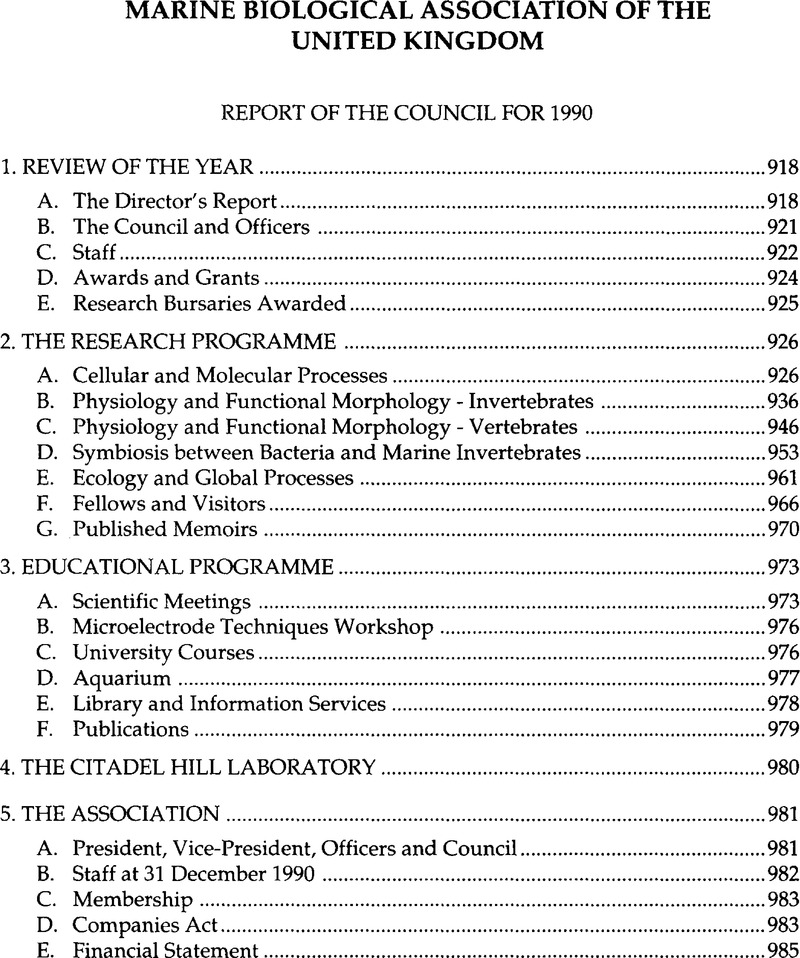The image is a photo of a table of contents page from a book titled "Marine Biological Association of the United Kingdom Report of the Council for 1990." The table of contents outlines five main sections, each with various subcategories. It begins with "Review of the Year" with subcategories A to E, numbered pages starting at 918. The second section, "The Research Program," has subcategories A to G, discussing different areas of research and their respective page numbers. The third section, "Educational Program," includes subcategories A to F covering different educational activities. The fourth section is "The Citadel Hill Laboratory," and the fifth section, "The Association," details organizational information with subcategories A to E. The page numbers range from 918 to 985, indicating it might be part of a larger compilation. 

**Table of Contents:**
1. **Review of the Year** ......918
   - A. Directors Report ......918
   - B. Council and Officers ......921
   - C. Staff ......922
   - D. Awards and Grants ......924
   - E. Research Bursaries Awarded ......925

2. **The Research Program** ......926
   - A. Cellular and Molecular Processes ......926
   - B. Physiology and Functional Morphology Invertebrates ......936
   - C. Physiology and Functional Morphology Vertebrates ......946
   - D. Symbiosis Between Bacteria and Marine Invertebrates ......953
   - E. Ecology and Global Processes ......961
   - F. Fellows and Visitors ......966
   - G. Published Memoirs ......970

3. **Educational Program** ......973
   - A. Scientific Meetings ......973
   - B. Microelectrodes Techniques Workshop ......976
   - C. University Courses ......976
   - D. Aquarium ......977
   - E. Librarian Information Services ......978
   - F. Publications ......979

4. **The Citadel Hill Laboratory** ......980

5. **The Association** ......981
   - A. President, Vice President, Officers, and Council ......981
   - B. Staff at 31 December 1990 ......982
   - C. Membership ......983
   - D. Companies Act ......983
   - E. Financial Statement ......985